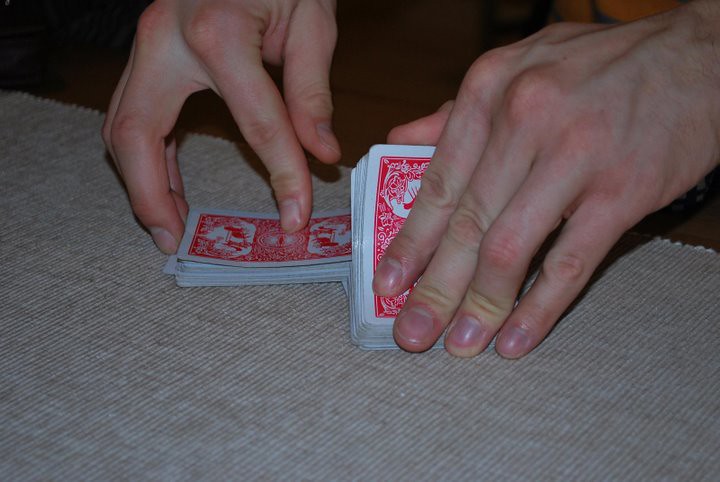In the photograph, a pair of distinctly Caucasian male hands are captured mid-motion while shuffling a deck of cards. The hands, characterized by their slender fingers, likely belong to an individual in their 20s or 30s. The deck, adorned with a red back featuring an intricate design of a man driving a horse-drawn wagon, is split between the hands, each holding a stack of cards facing opposite directions. Beneath the hands, a white-gray tablecloth covers a brown wooden table. A small stack of black-and-white poker chips peeks out from under the left hand, adding a touch of intrigue to the scene.